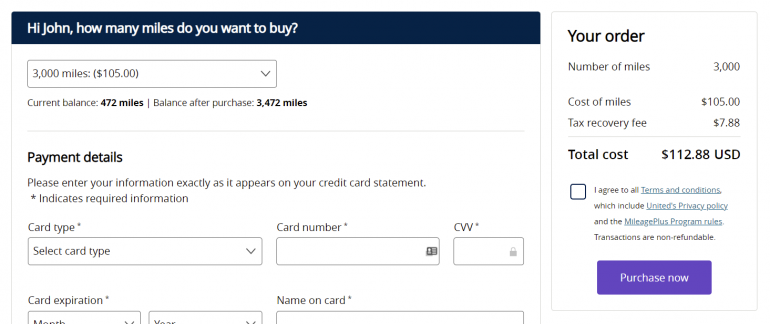Detailed webpage screenshot description:
 
The screenshot portrays a user interface designed for purchasing airline miles. The layout is divided into two distinct sections.

The left section, which is horizontally oriented, features a black top bar with white text greeting the user: "Hi John, how many miles do you want to buy?" Below this is a white background populated with interactive elements. The central component is a drop-down menu, currently set to 3,000 miles, priced at $105. Directly below the drop-down are statements displaying the "Current Balance: 472 miles" and "Balance After Purchase: 3,472 miles." 

Further down, there is a "Payment Details" section prompting users to input their credit card information exactly as it appears on their statements. Required fields include Card Type, Card Number, CVV, Card Expiration, and Name on Card, each paired with respective text boxes.

The adjacent, vertically-oriented right section provides a compact summary of the order within a white box edged with a gray border. Titled "Your Order," this section lists:
- Number of Miles: 3,000,
- Cost of Miles: $105,
- Tax Recovery Fee: $7.88,
- Total Cost: $112.88.

At the bottom of this summary is a checkbox to agree to terms and conditions, followed by a prominent "Purchase Now" button enabling the completion of the transaction.